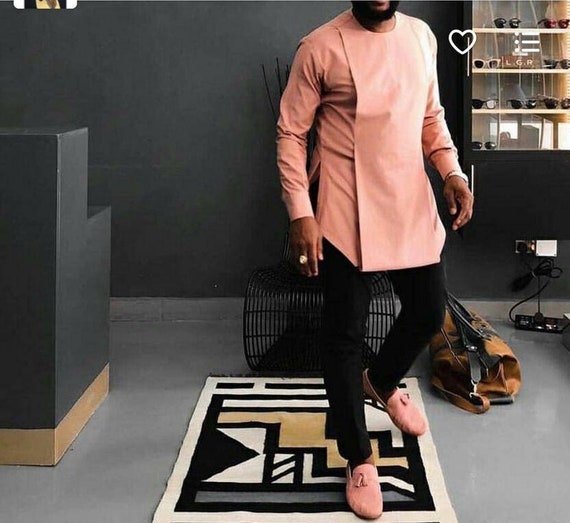The image depicts a man standing inside a modern environment, likely a shop where sunglasses are sold, indicated by the display case of various sunglasses in the top right-hand corner labeled with the letters "LGR." The setting features a black wall in the background. To the left, there's a black counter with a small brown base. Positioned on the black and white geometric-patterned rug, which also includes brown and white details within a white edge, the man sports dark skin and a distinctive black beard that outlines his jawline and chin. He is dressed in a long-sleeved, salmon-colored shirt with a vertical flap of the same material, black pants, and matching salmon-colored shoes. His outfit, reminiscent of traditional Indian attire, has a slightly robe-like appearance. Around his right hand, he wears a ring. Behind him, there is an industrial black fan and what seems to be a grayish-brown leather satchel or tool bag. The general ambiance of the space and the man's attire suggest a blend of modern and traditional elements.